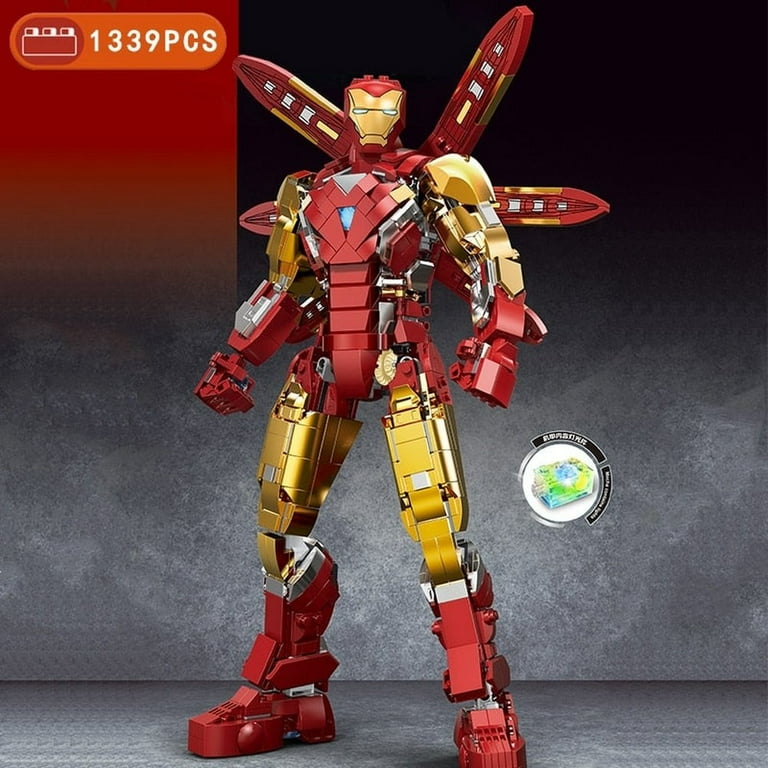The image depicts a square picture of an Iron Man action figure, who is a well-known Marvel superhero. The figure is wearing a red robotic suit accented with gold. Notably, the thighs, forearms, shoulder to elbow sections, and face plate are all gold, while the rest of the suit is predominantly red, including the head and lower legs. Iron Man is standing upright against a gray, concrete-like background that transitions to black in the upper right corner. The intricate suit design also includes blades attached to its back, with five tips visible in red and gold.

Iron Man's legs are primarily red with gold upper legs and silver knees. The propellers on his back further enhance his robotic appearance. In the upper left corner of the image, there's a label featuring a red oval with the text "1339 PCS" in white, indicating that the figure is made out of 1339 snap-on pieces akin to Lego bricks but potentially an off-brand. Near Iron Man's right thigh, a circular element with blue and green colors emits a shining effect, adding to the visual complexity of the image.